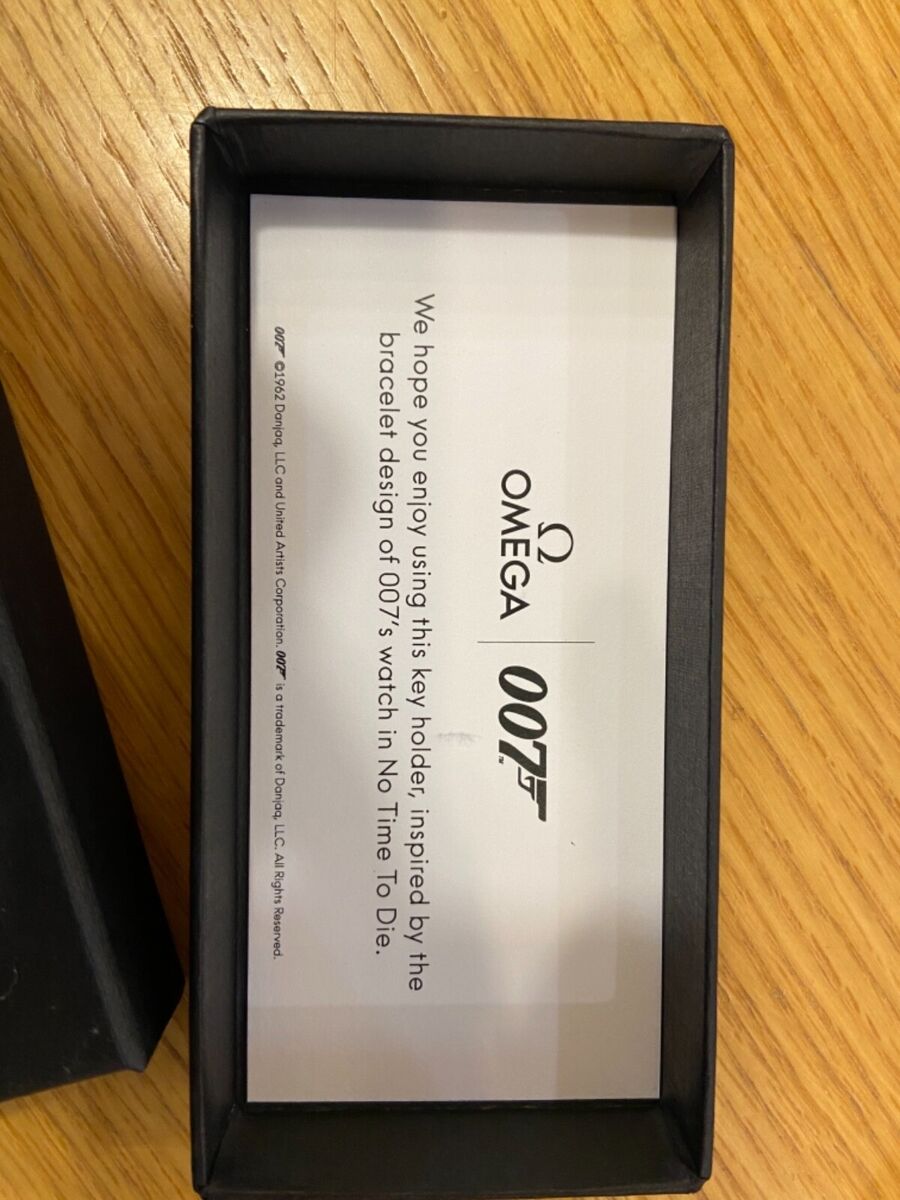The image depicts a close-up of a white rectangular paper with black text that reads, "Omega 007. We hope you enjoy using this key holder inspired by the bracelet design of 007's watch in No Time to Die." This paper is part of a black case or holder, which is open with its cover lying next to it. The case and paper are placed atop a brown wooden or possibly Formica table, under bright natural lighting, highlighting the clear and crisp details of the setting.